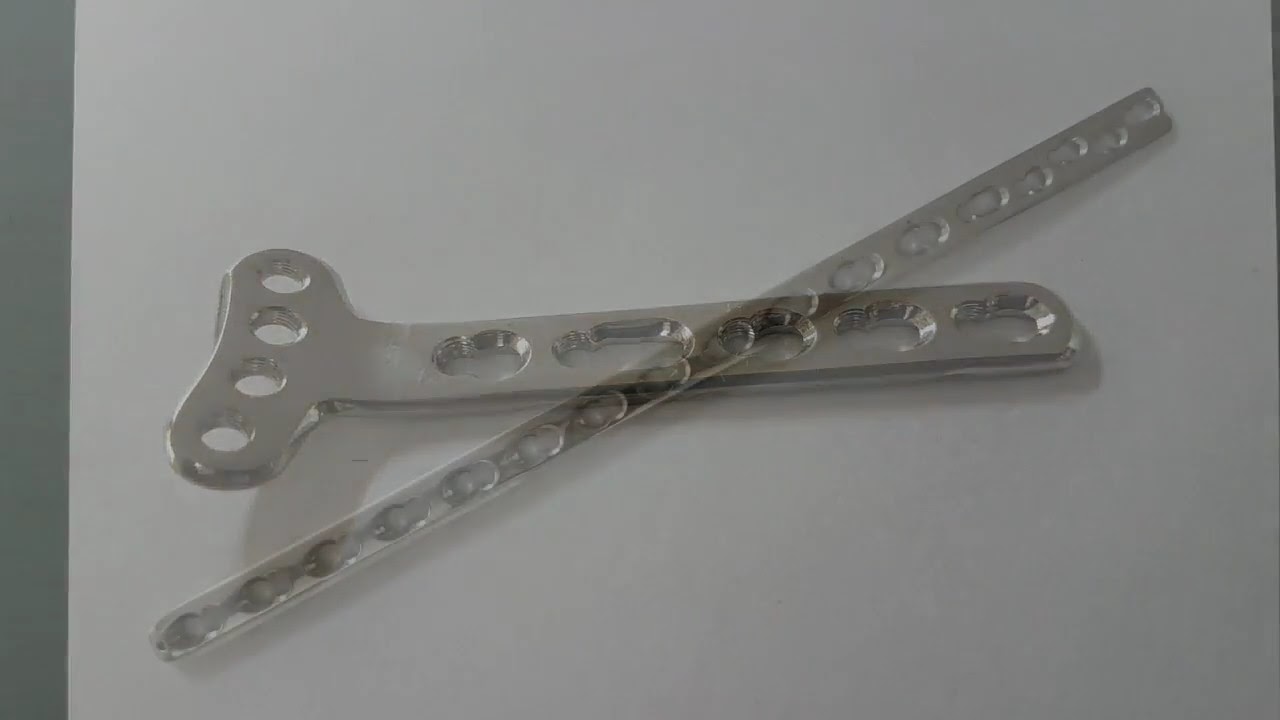The image features two metallic instruments set against a white sheet background. The instruments, both silver in color, intersect each other, with one lying horizontally across the other, forming a T-shape. The horizontal tool is wider and features four holes across its top and additional holes along its length. The vertical tool is slimmer and positioned at a 45-degree angle under the horizontal tool, also having numerous smaller holes along its body. Both tools appear somewhat translucent and slightly blurred, indicating potential image editing effects. A vertical gray strip runs along the left side of the image, adding contrast to the otherwise white background. The image has no text and appears to be a generic stock photo of two intersecting tools.